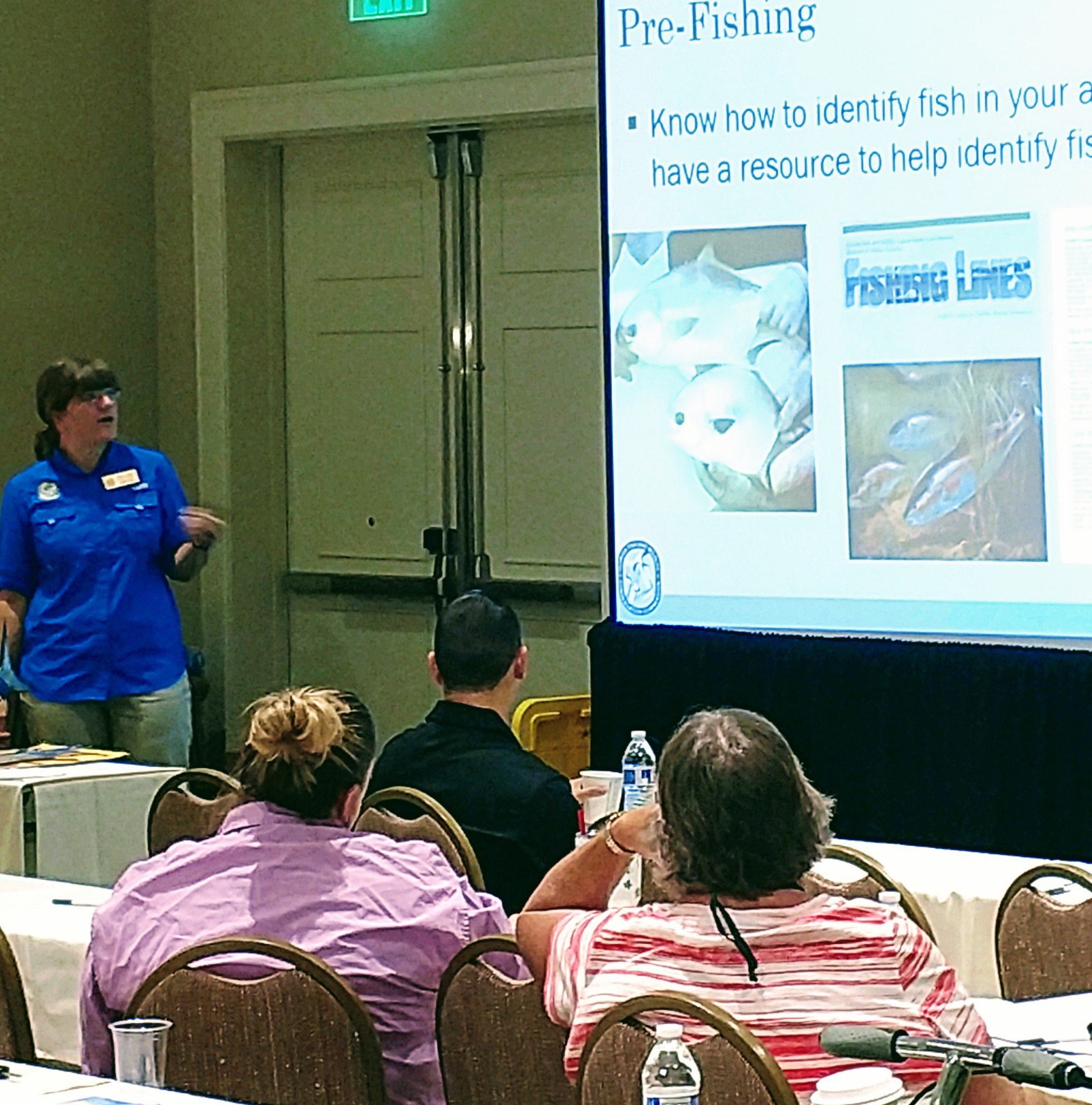In this image, a woman is delivering a lecture in what appears to be a classroom or meeting hall, with light brown or cream-colored walls and white double doors marked with a green "Exit" sign in the background. The instructor is a Caucasian woman with black hair pulled back into a ponytail. She is wearing a blue blouse, khaki pants, a gold name tag, and glasses. Her hand is animated as she engages with the audience. Behind her, a large projector screen displays a PowerPoint slide that reads "Pre-fishing: Know how to identify fish in your A..." (with part of the text cut off), followed by "have a resource to help identify FIS..." and two pictures of fish with captions mentioning fishing lines. In front of the instructor, three attendees sit on chairs at tables covered with white tablecloths, each with water bottles in front of them. One female attendee wears a purple shirt and has a ponytail, another woman is in an orange and white striped shirt, and a man sits ahead of them wearing a black shirt. All three are focused on the screen, attentively following the presentation.